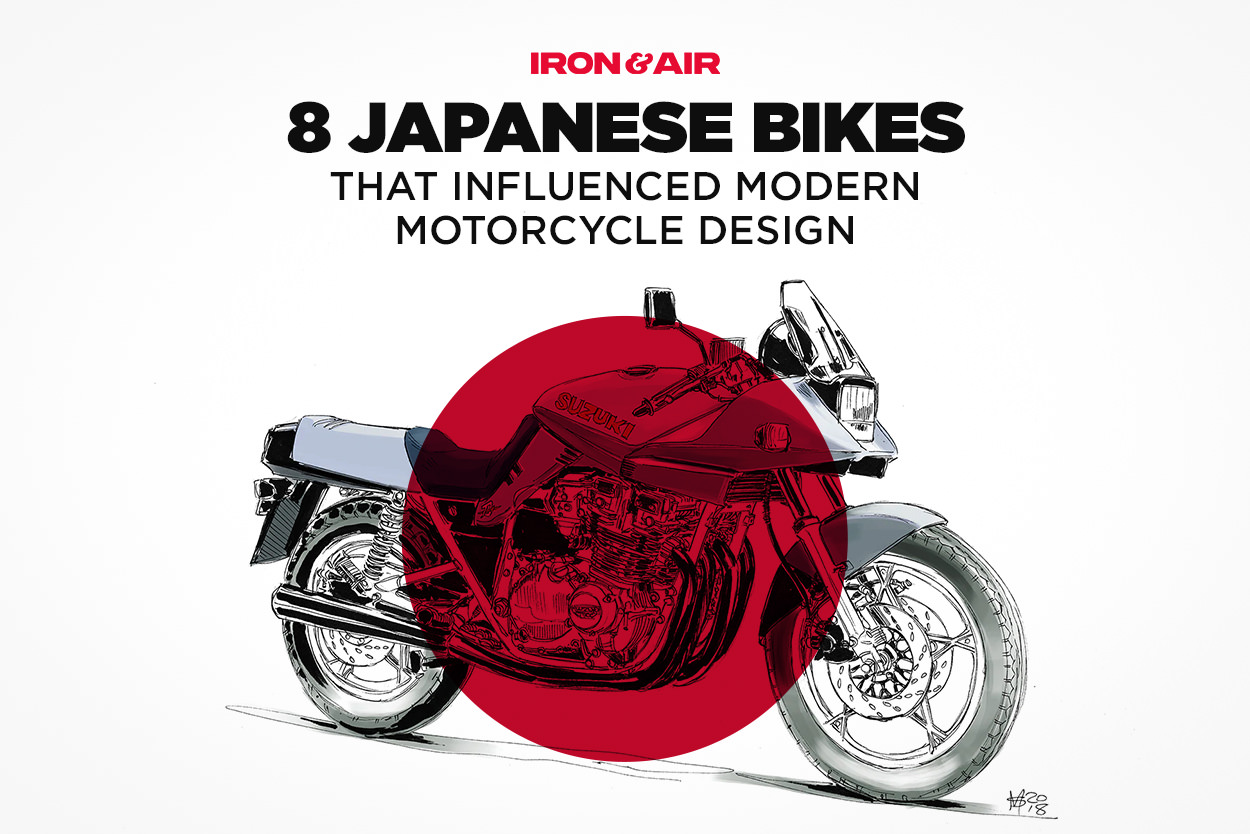The image appears to be a front cover advertisement for a magazine titled "Iron and Air." The magazine's title, "Iron and Air," is prominently displayed at the top in bright red, capital letters. Below this, in bold capital letters, it reads "Eight Japanese Bikes That Influenced Modern Motorcycle Design," with "Eight Japanese Bikes" significantly larger than the rest of the text. The background of the image is light gray with a black and white, hand-drawn Suzuki motorcycle prominently featured in the lower middle of the image. A large red circle overlays the center of the motorcycle, reminiscent of the Japanese flag, drawing attention to the word "Suzuki" on the bike. The motorcycle illustration includes subtle gray and white details. The artist's autograph, dated 2018, is visible in the bottom right corner of the image.